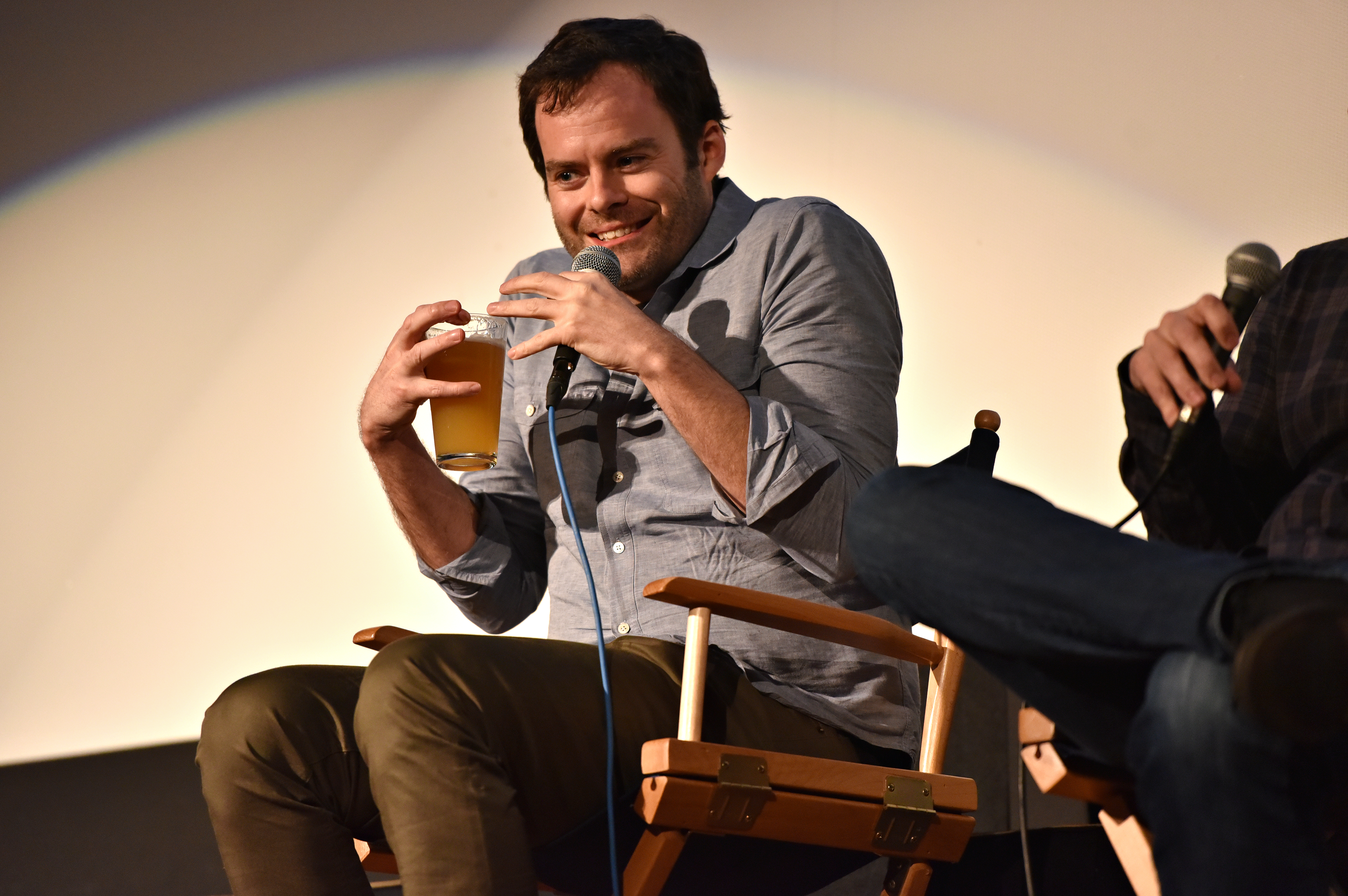The image depicts a man seated in a director's chair with wooden armrests, set against a background of a white wall with shadowy details and a blue arch of light. The man, clad in a gray button-down collar shirt and tan pants, is scrunching his shoulders and bending his elbows while holding a beer or orange juice in his right hand and a wired microphone with a blue cord in his left. He is engaged in conversation or addressing an audience. Next to him, there is another person whose face is out of the frame, visible only from their upper shirt and blue jeans with their right leg crossed over their left knee. This second individual, wearing a brown plaid shirt, is also holding a microphone, indicating that both are likely participating in a panel or discussion.